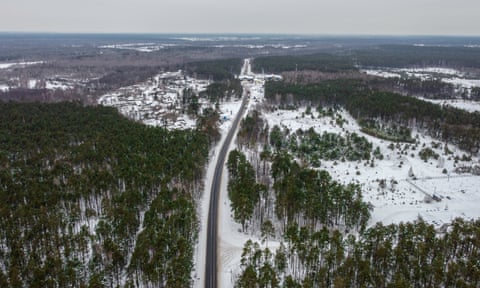This aerial image, captured from above, depicts a serene winter landscape with a gray sky. The central focus is a two-way highway running vertically through the middle of the scene, extending almost to the horizon where it fades out of view. Snow blankets the ground, creating a stark contrast with patches of brown dirt and areas where forests seem to have died or been burned, leaving behind gray or blackened timber. Green pine trees frame the foreground and right-hand side, adding a touch of color to the otherwise muted palette. Midway back, you can see power lines stretching left to right. No vehicles are present on the road, and the overall setting is devoid of human activity. Toward the horizon, the landscape transitions into distant water or mountain formations, slightly blurred by the overcast weather.